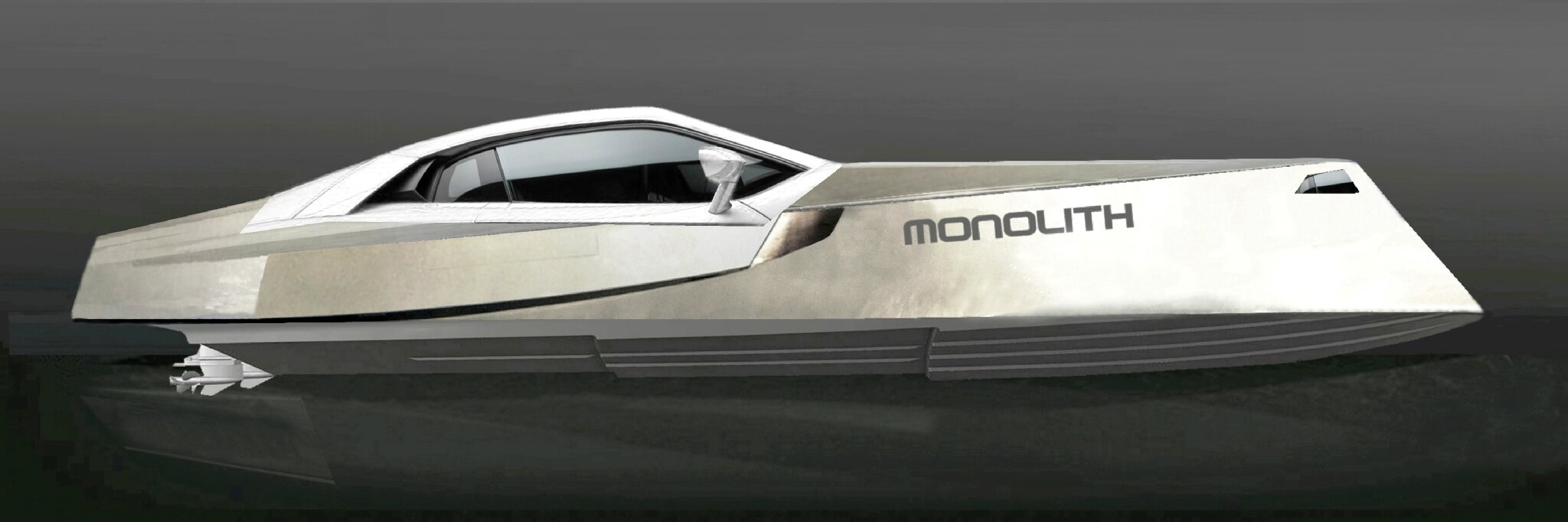The image showcases a sleek, futuristic speedboat rendered in CGI, with a design reminiscent of the Tesla Cybertruck's stainless steel aesthetic. The boat, taking on a silverish-bronze hue with elements of white and gray, features a distinctly aerodynamic structure. Its sharp, angular lines are prominent along the sides and front hood, embedding it with a sense of motion even while stationary. The front hood houses a rectangular cutout, and the left side sports another hole, possibly serving as an exhaust. The brand name "Monolith" is inscribed on the front right side of the hood. The boat is equipped with blacked-out windows, a roof that angles upward before dipping, and car-like rearview mirrors affixed to the sides. At the back, a white rotor with gray fans hints at its high-speed capabilities. The setting is minimalistic, with a calming gray gradient background and a subtle reflection underneath, suggesting it's gracefully resting on water.